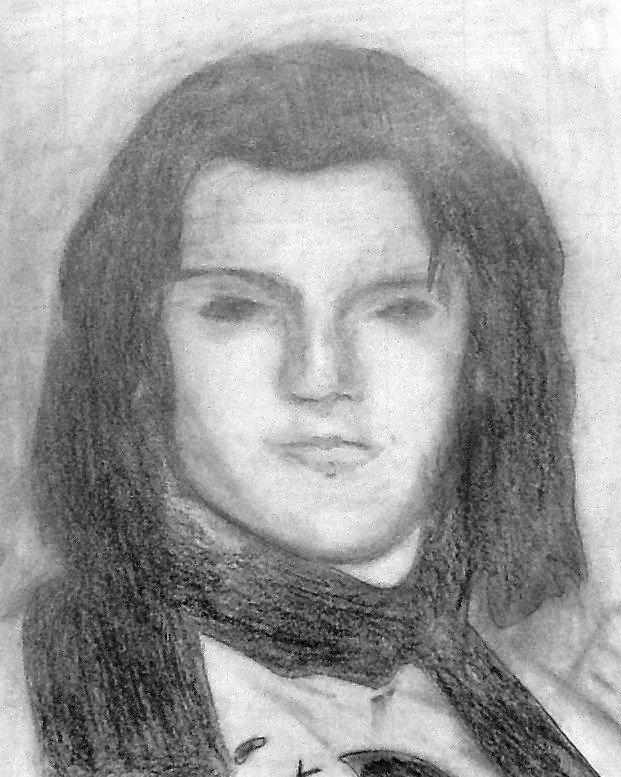The image is a black and white pencil drawing of a man with shoulder-length, straight hair that is dark with lighter gray streaks due to the shading of the pencil. His hair is asymmetrical; the left strand extends slightly past his shoulder, while the right strand stops at the shoulder. He has a broad nose, thin lips, and deep, darkly shaded eyes with equally dark eyebrows. His lips are outlined in a darker gray. The man is wearing a scarf that wraps around his neck and over his shoulders, with the left side of the scarf appearing lighter in gray due to shading techniques, creating a contrast with the white of the paper. Some hair falls into his face near his eye. He also appears to be wearing a shirt with many creases, depicted through varying shades of gray and darker black. The drawing is set against the white paper, accentuating the contrast between the man's white face, dark hair, and black scarf. The man's body is slightly tilted to the bottom right, and he is staring directly in front of him, giving a detailed yet not overly intricate portrayal.